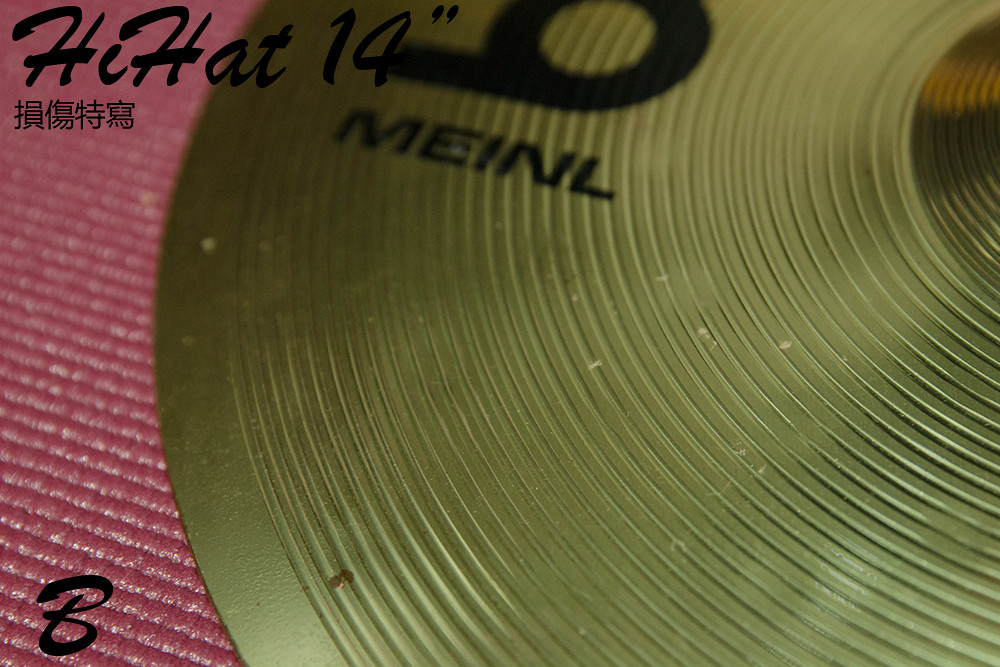The image shows a close-up of a 14-inch hi-hat cymbal situated on a pink, horizontally-striped textured background, possibly a cloth or tablecloth with a decorative design. The cymbal is gold in color with a copper-hued center ring. The word "MEINL" is prominently written in black cursive at the top, along with additional Asian text directly below it. The lower left corner of the cymbal features a black letter 'B' in the same cursive style. The cymbal surface exhibits some specks, including white specks in the middle, a couple on the outside, and a brown speck on the left-hand side, indicating it has been used. The image is framed to display only a portion of the cymbal, emphasizing its texture and markings.